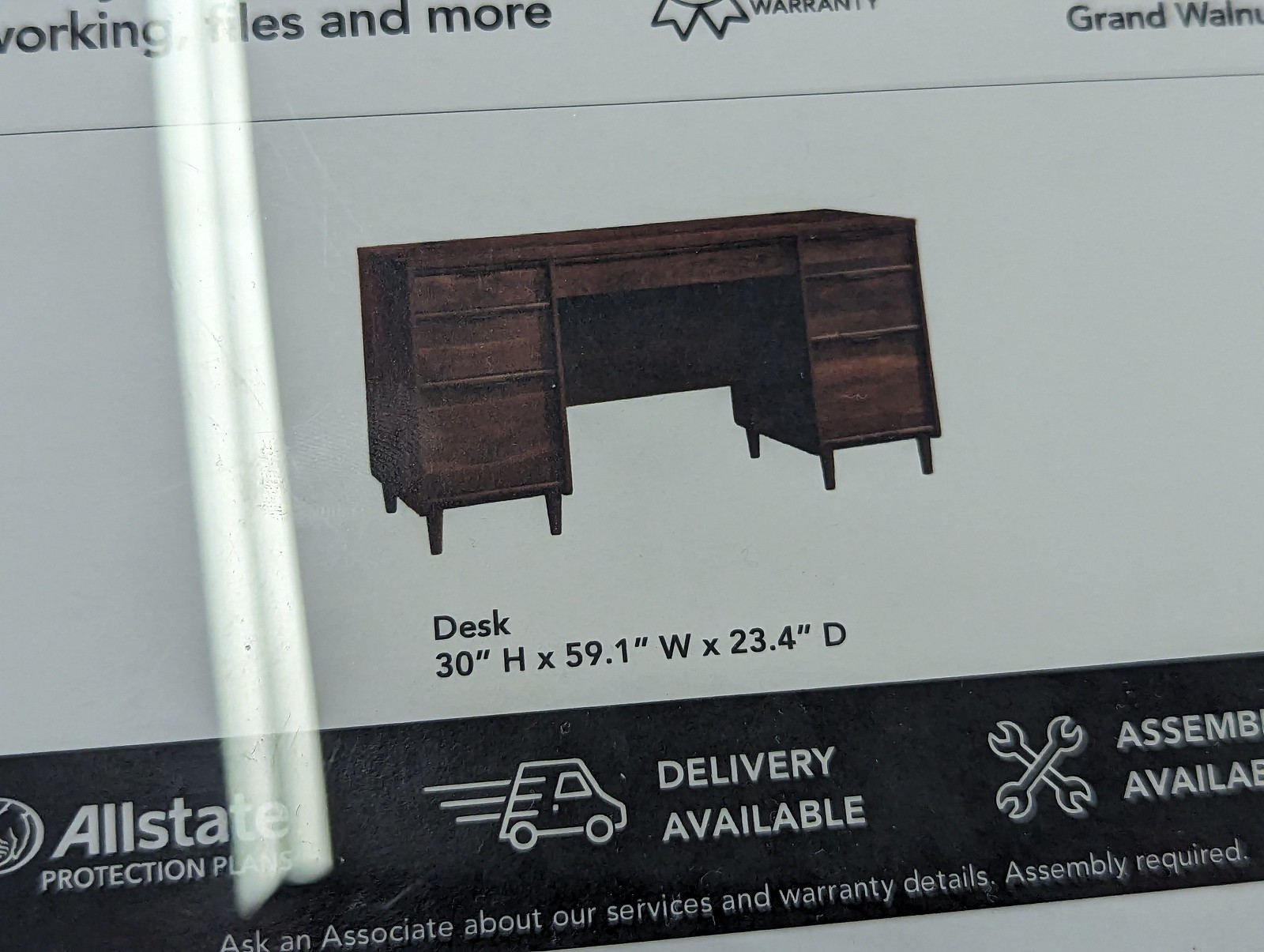The image appears to be a portion of a catalog page or product packaging showcasing a brown wooden office desk. The desk measures 30 inches high by 59.1 inches wide by 23.4 inches deep. It features peg legs and includes a central leg space flanked by three rectangular drawers on each side of the writing surface. Below the desk's image is descriptive text listing its dimensions. A black footer band beneath this text provides additional information: "All State Protection Plans," "Delivery Available," and "Assembly Available," each accompanied by respective icons—a shield, a sketch of a delivery van, and crossing wrenches. Further down, the text advises, "Ask an associate about our services and warranty deals. Assembly required." The overall image is slightly tilted counterclockwise with a vertical glare on the right side. Partial text towards the top mentions "working tiles" and possibly "walnut," indicating additional details that are partially cut off.